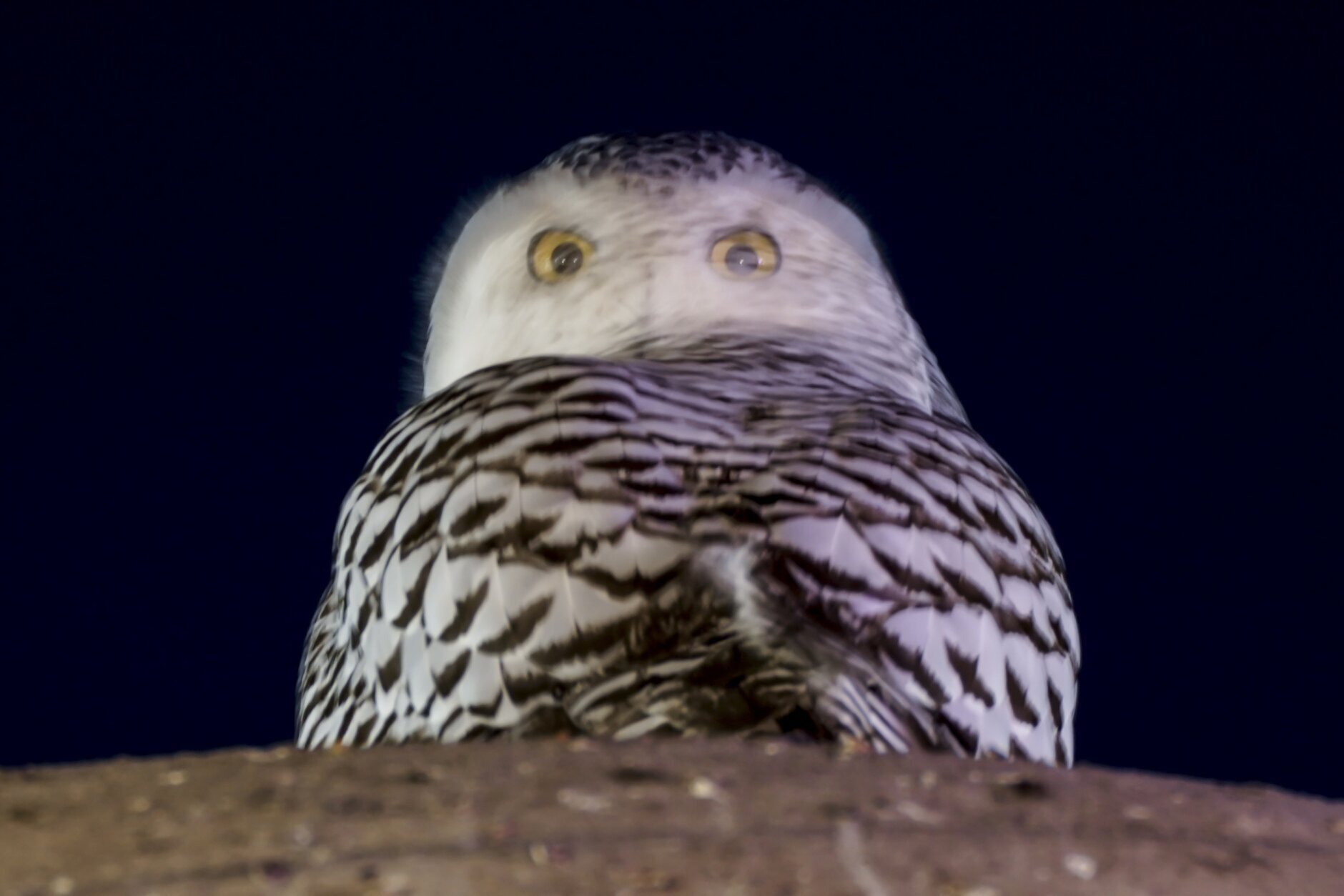This outdoor nighttime photograph, measuring approximately five inches wide and four inches high, captures a striking image of a snowy owl. The foreground features a dark brown structure resembling a tree branch or stump, embellished with specks of black and white. This could be the owl's perch. Above this, the background is a black sky, enveloping the primary subject: a snowy owl. The owl's body is predominantly white with touches of black, especially around the feathers on its wings and tail. Its head, seemingly blurred from a swift motion, is turned towards the camera, revealing a face framed by soft white feathers with traces of black. Two large, round yellow eyes with dark centers dominate the owl’s face. The photograph, taken from a low angle as if from the ground up, emphasizes the owl's downward gaze, lending an ethereal and intense focus on the viewer.